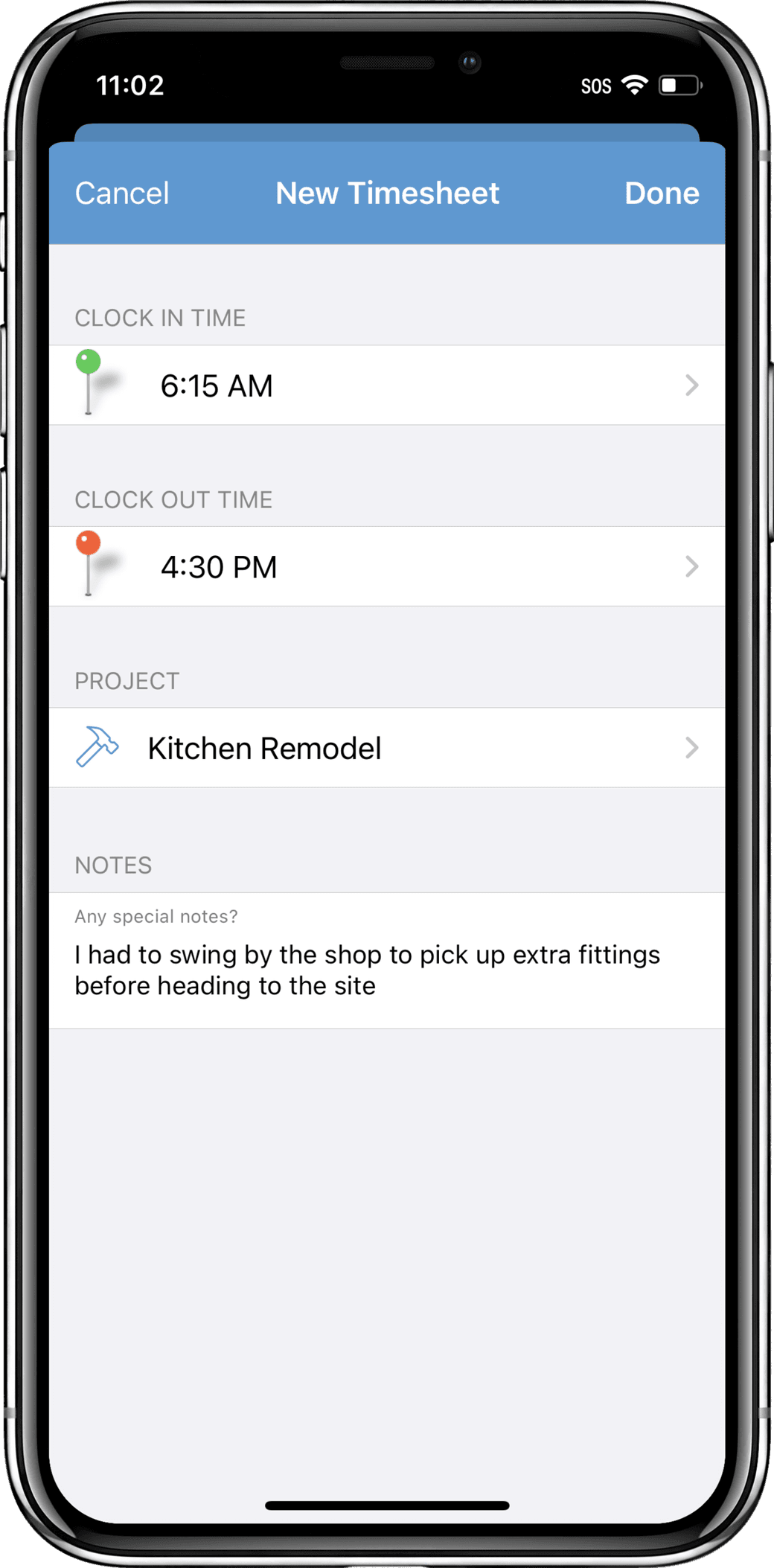This is a detailed mock-up of an iPhone, showcasing its various elements with crisp clarity. The sleek device is adorned with a shiny silver band along the edge, complemented by a faux shine on the glass surface. The image appears to be a meticulously designed digital rendition, possibly created using Illustrator or another CGI tool. 

At the top, the black status bar displays key icons: a small camera icon indicating the presence of a front-facing lens, the time reading 11:02, an SOS signal, a Wi-Fi indicator, and a battery level showing approximately 40% charge. Below this bar, a blue section is partially obscured by a pop-up window that likely slides up from the bottom.

The pop-up window features a blue header with options to "Cancel," "New Time Sheet," and "Done." Inside the window, the first line on the left reads "Clock In Time" with a green pin icon, which casts a subtle shadow. The time displayed next to this is 6:15 AM. Beneath it, "Clock Out Time" is indicated with a red pin icon and the time shown is 4:30 PM. These entries have arrow icons to their right for further interaction.

The third section is labeled "Project," featuring a hammer icon and the text "Kitchen Remodel." This is followed by a grey bar. Further down, there is a section labeled "Notes" asking, "Any Special Notes?" Below this prompt, text has been typed in, stating, "I had to swing by the shop to pick up extra fittings before heading to the site." 

A thin green line underlines this note, contrasting against the white background. The bottom of the screen is marked by a centered black line, completing the clean and precise design of the mock-up.